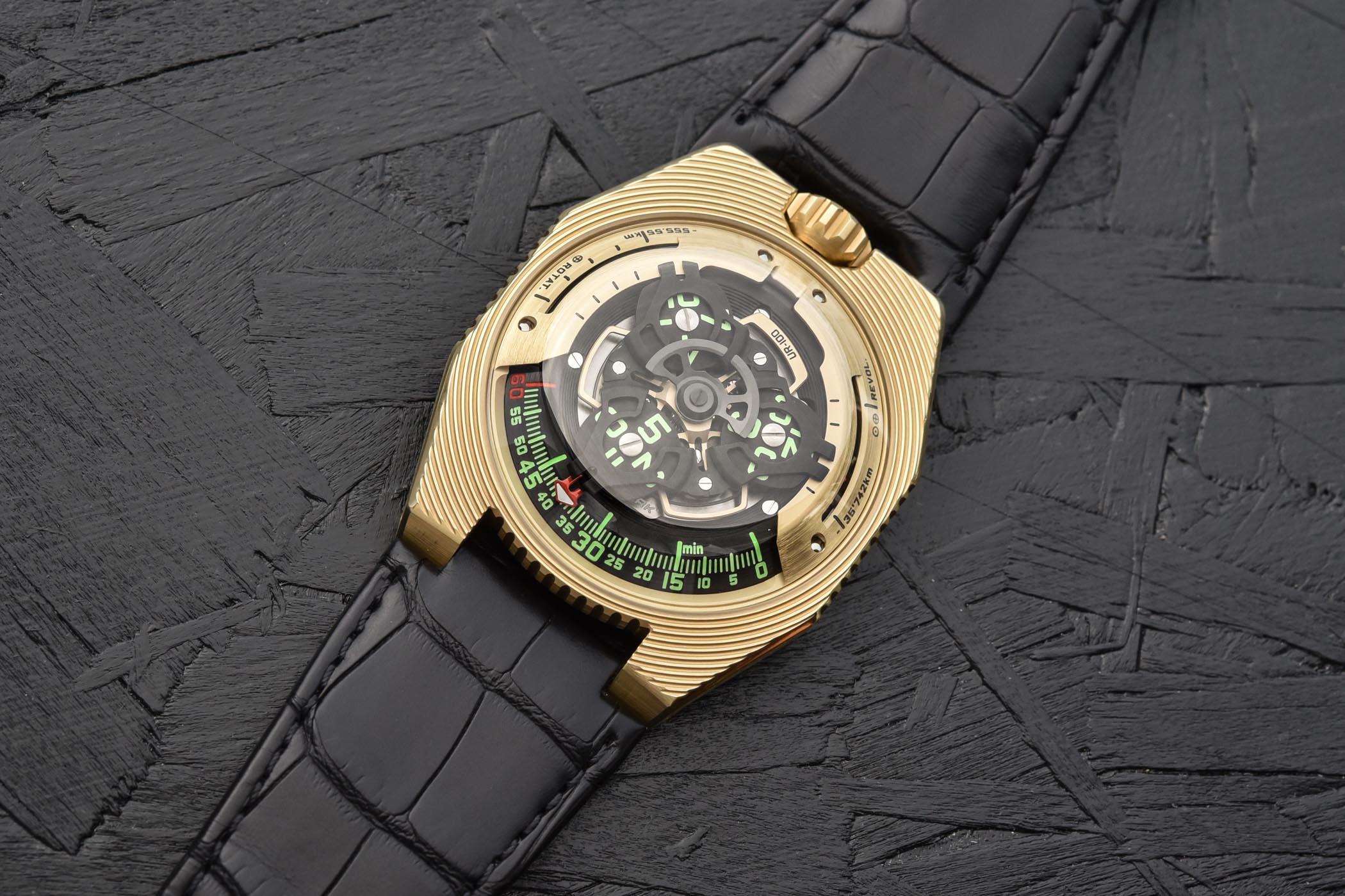The photograph captures a luxurious gold wristwatch with a black alligator-patterned leather band, set against a black particle board background. The watch is displayed diagonally across the center of the image, tilting upward to the right. Its intricate gold face showcases visible internal gears, framed by concentric gold circles that enhance its high-end appearance. The black leather strap features a distinctive rectangular pattern, resembling a turtle shell design. Positioned at the bottom of the watch face is a green scale dial with a red arrow pointing to the number 40, possibly indicating a compass or barometric measurement. The gold winding knob is located at the top, adding to the watch’s sophisticated detail. The overall image is clear and well-lit, highlighting both the watch's craftsmanship and the textured particle board beneath it.